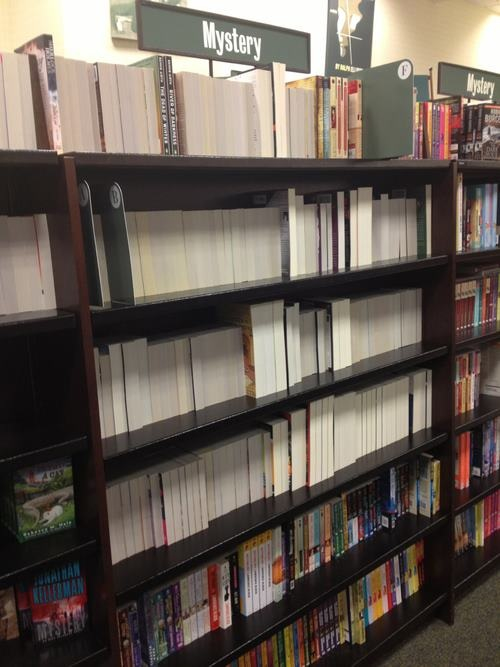This detailed photograph captures a section of a bookstore, specifically in the mystery genre area. The image prominently features a black and brown wooden bookshelf with six levels of shelves. The bottom two shelves are filled with a variety of colorful paperback books, correctly oriented with their titles visible. In contrast, the top four shelves display books with their pages facing outward, obscuring their titles for an unknown reason. Above the top shelf, there is a prominent horizontal gray sign with the word "Mystery" in white letters, indicating the genre section. Flanking this central bookshelf are the edges of two additional bookshelves on the left and right sides of the image, both also marked as part of the mystery section with similar gray signs featuring white text. The right side of the image reveals a section divider with the letter "F," while the background shows an off-white wall adorned with a black-and-white poster. The bookstore floor is covered with a gray carpet. This composition captures the organized yet slightly chaotic nature of the mystery section in this bookstore.